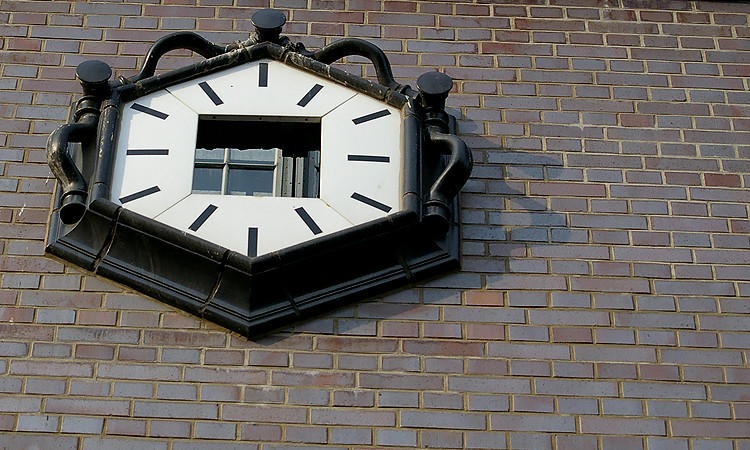This image showcases a striking and unique clock mounted on an exterior brick wall, which appears to be part of an old factory or public building, suggesting historical and functional significance. The clock, either octagonal or hexagonal in shape, is framed with black metal, giving it an industrial aesthetic. The face of the clock is white, featuring black dashes in place of numerals, with bold black hands for easy readability. One of the most distinctive features is a square cut-out in the center of the clock, through which a four-paned window on the wall can be seen. Surrounding the clock, black metal elements, resembling handles or pipe-like structures, add a decorative touch and might play a role in mounting or operation. The brick wall behind the clock is composed of reddish-brown bricks with a slight variation in tone, offering a rich texture and color contrast that enhances the visual appeal of the image.